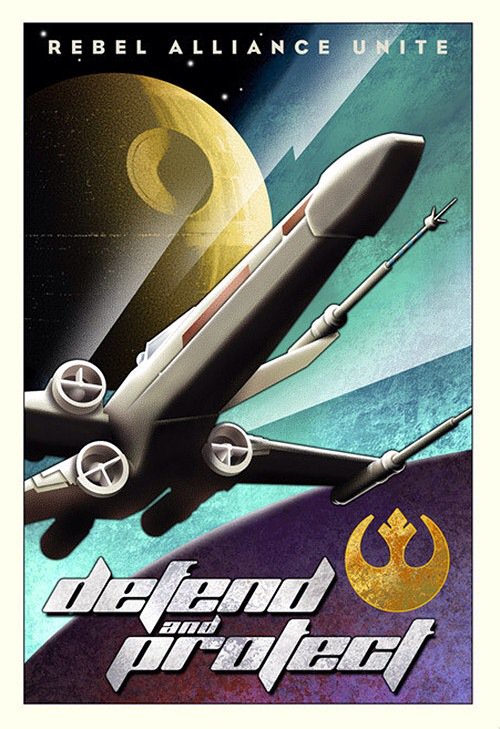The poster is a detailed and vibrant vertical rectangular image showcasing a futuristic B-wing spaceship, flying diagonally from the lower left to the upper right. The silver spaceship, adorned with ion cannons on its wings and engines around its base, is set against a deeply black, star-studded space backdrop with white dotted stars. Dominating the middle background is a depiction of a yellow Death Star with a pronounced indent, characterized by both light blue and green diagonal stripes extending from its lower section. 

At the very top of the poster, the bold white text reading "Rebel Alliance Unite" captures attention, while at the bottom, the phrase "Defend and Protect" stands out in large lowercase white letters. Situated above the word "Protect" is the gold Rebel Alliance symbol, which resembles a crown atop a three-quarters filled circle with additional intricate detailing. The overall composition and the intertwining elements emphasize the call to action for unity and defense among the Rebel forces in a vividly futuristic and space-oriented setting.